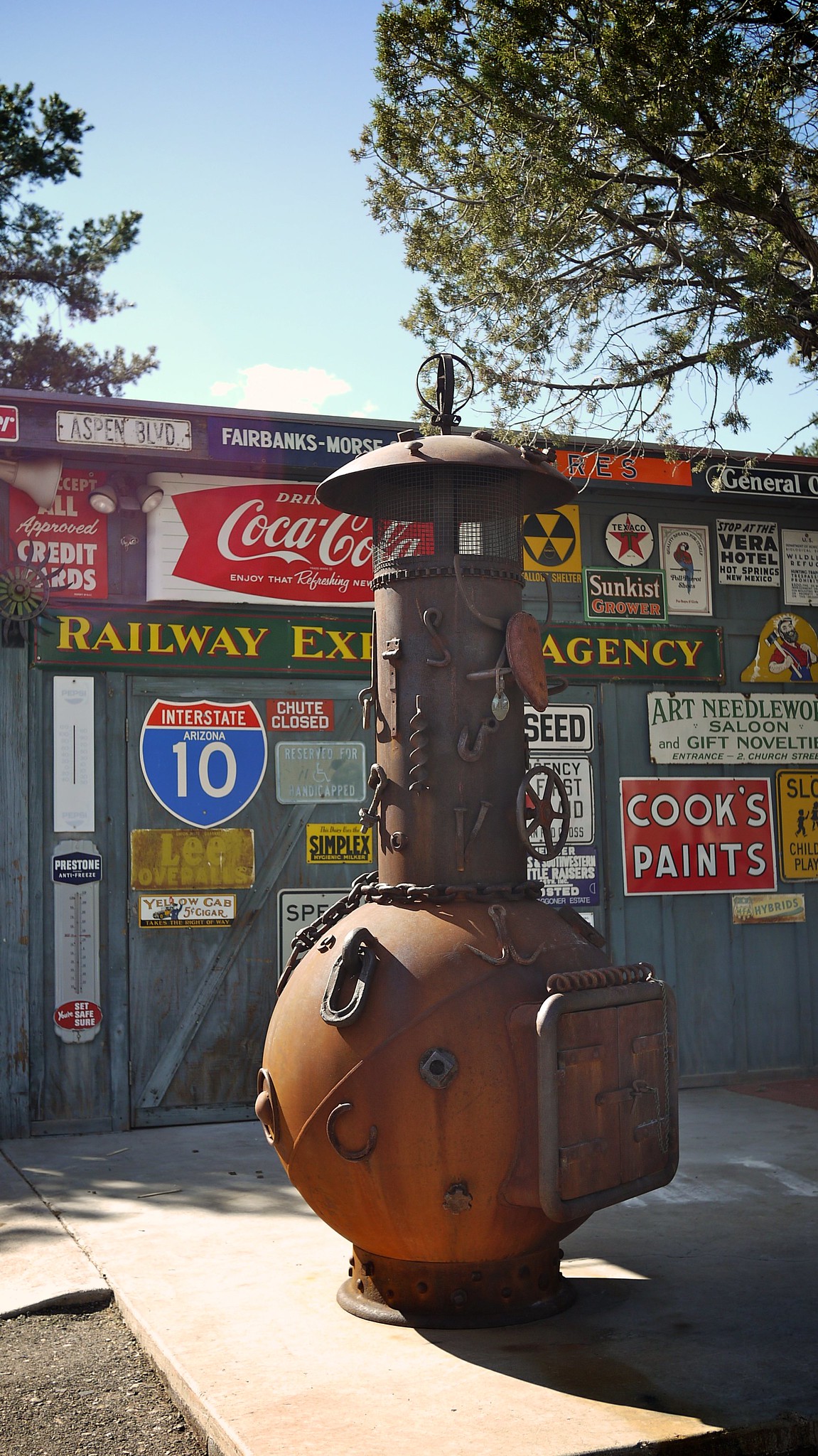In this outdoor photograph, a striking metal sculpture resembling an old pot-bellied stove or meat smoker sits prominently on a flat concrete surface, likely part of a walkway or driveway. This rust-covered sculpture features a bulbous, circular body with a double door at the front for loading, and an extended tube-shaped chimney or vent at the top. Various horseshoes, hooks, and welded tools intricately adorn its surface. Despite its rustic appearance, the large sculpture stands nearly as tall as a person, emphasizing its commanding presence.

Behind the sculpture, the backdrop consists of a weathered gray wooden shed building adorned with an assortment of vintage tin signs. Notable signage includes "Cook's Paint" in white letters on a red background, a classic Coca-Cola ad, and an Interstate 10 Arizona marker. The shed’s collection of signs adds a nostalgic ambiance to the scene. 

The sky above is a light blue sprinkled with fluffy white clouds. Overhanging branches covered in light green leaves peek from the top of the image, adding a touch of natural beauty. Sunlight from the left casts shadows toward the right, highlighting the textures and details of the metal sculpture and the old building, creating a warm, inviting atmosphere on this sunny day.